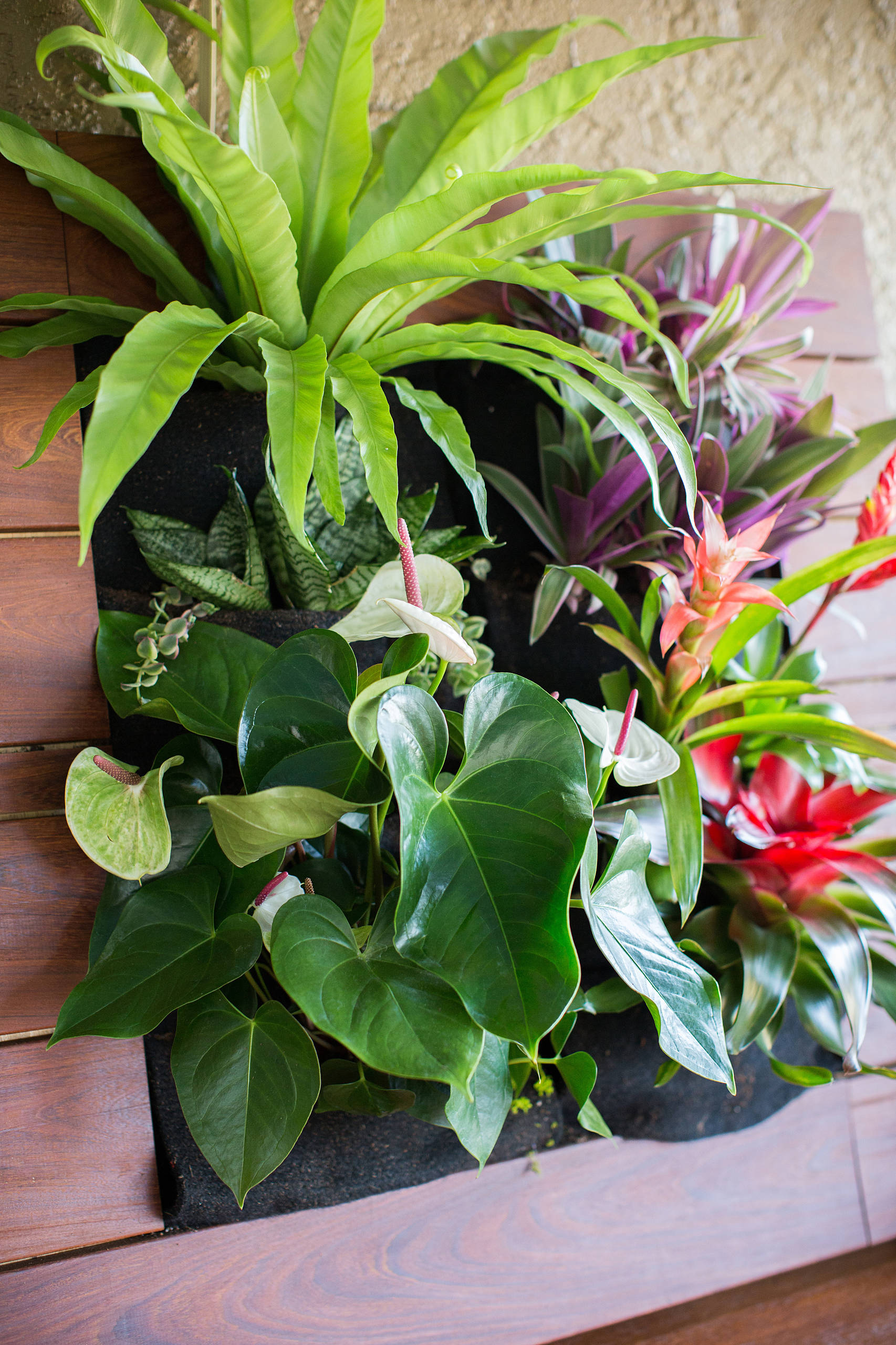The image depicts a vibrant array of plants and flowers arranged within a wooden planter, which is crafted from honey-colored wood slats forming a square shape. This planter is bordered with wood panels and is set against a textured, non-smooth concrete or stucco wall, while the floor beneath it is a medium brown color. Inside the planter, landscape fabric or felt supports the various plants, which include more than four different kinds. On the bottom left, there's a plant with red flowers, while on the bottom right, another set of red flowers can be seen. In contrast, the bottom left also hosts a plant with white flowers featuring pink stems. The top left showcases a plant with long, light green leaves fanning out, giving a crowning effect. On the top right, there are plants with purplish leaves and some flower buds. Small plants with green and light green striped leaves are interspersed among these larger plants. Additionally, there's mention of a flower resembling an anthurium among the mixed varieties, which include flowers of pink, purple, and reddish hues, as well as one described as having white petals with a warm, vertical pink interior. All these diverse plants and flowers are closely packed into the central space within the planter, creating a lush, detailed display.